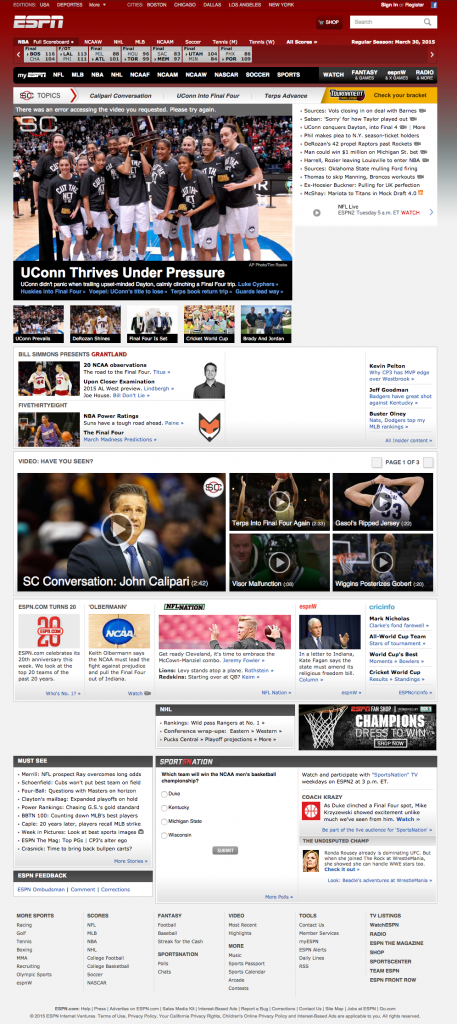This is a screenshot of the SESPN website showcasing three different pages. On the first page, the primary story is titled "Yukon Thrives Under Pressure." It features a women's sports team celebrating their victory. The team members are dressed in grey short-sleeved t-shirts and white shorts, with white lettering and a shield emblem on their t-shirts. They are indoors on a sports court, posing with a trophy amidst the backdrop of spectators seated in the stands. Additionally, the website highlights various news stories including an interview with John Calipari, likely a sports coach from SC. Another featured section appears to be dedicated to basketball-related news stories.